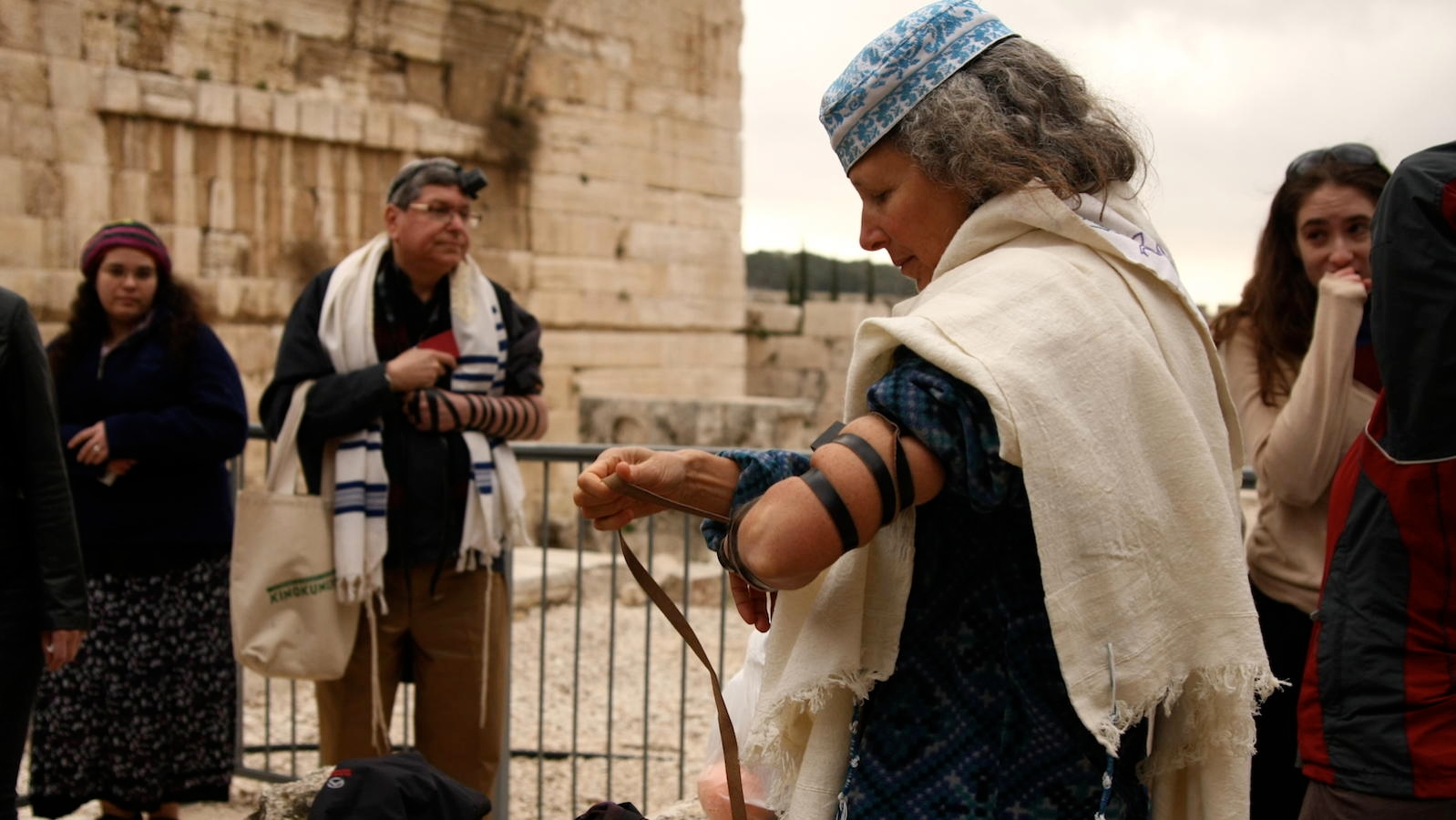In this photograph, a group of six people is gathered in front of an ancient, water-stained stone building, likely in a historical or religious site, with metal barricades in the background. The central figure, a woman with short blonde or grayish curly hair, is prominently featured in the foreground. She wears a blue ethnic cap and a white shawl over a blue outfit, and is binding her left forearm with black or leather strapping using her right hand, suggesting an activity of religious or cultural significance. To her right stands a younger girl, smiling with her hand to her mouth, seemingly amused or engaged. Also visible is a man in the background draped in a white prayer shawl with blue horizontal stripes, wearing glasses and a small cap, possibly indicating he is Jewish. He looks towards the central woman. To his left, another woman in a red hat and black coat watches the photographer. The scene overall suggests a diverse group of individuals, potentially tourists or pilgrims, interacting in a significant and historical Middle Eastern locale.